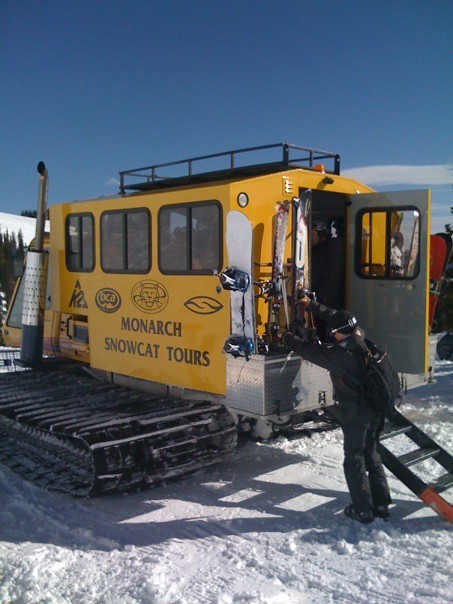This photograph captures a bright, sunny winter day with a vivid blue sky and abundant snow on the ground. At the center of the image stands a large, yellow snowcat machine, prominently displaying the words "Monarch Snowcat Tours" in black lettering on its side. The machine has tank-like treads, comparable to those found on tractors, extending from its body. It features a large, vertical exhaust pipe at the front, which is another noticeable element. 

A reflective sheen from the machine glistens on the snow, enhancing the clarity and brightness of the scene. The back door on the snowcat is open, revealing a set of small steps leading inside. Next to these steps, a woman dressed in a black ski outfit, including a hat, can be seen handling some snowboards, which are being stowed in the back of the vehicle. 

In the backdrop, a large snowy hill adorned with green trees unfolds, contributing to the picturesque mountainous landscape. Some additional details include a gray ladder with an orange tip emerging from the side of the snowcat and a black rack atop the vehicle. There is also a peculiar metal tool with a blue end, described as resembling an oversized giant toothbrush, positioned on the left-hand side. Off to the right, partially visible, another vehicle with red coloring appears. The scene suggests an inviting and adventurous atmosphere, ready for a snowy excursion.